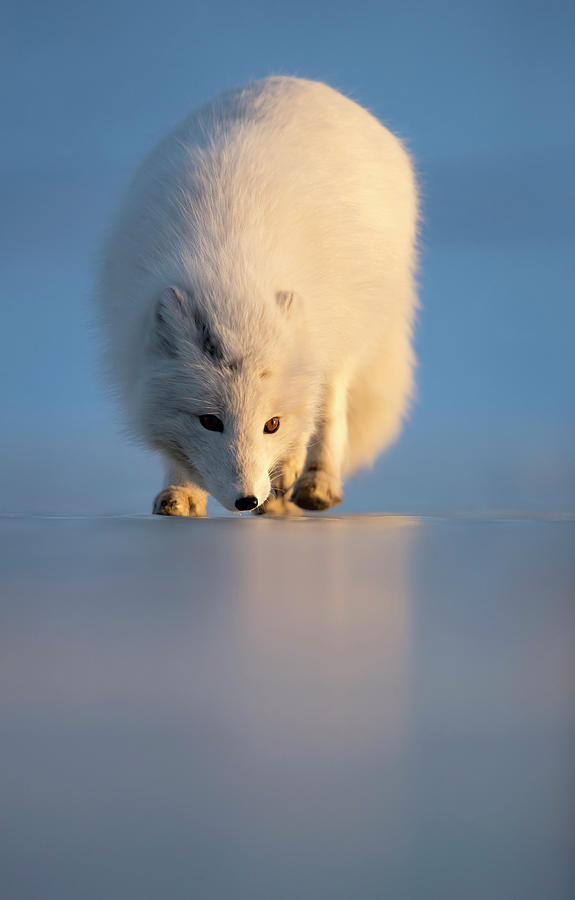The image features an Arctic fox, entirely covered in fluffy white fur, walking cautiously across an icy, reflective surface with a faint, hazy reflection below. The fox's small ears are positioned close to its head, and it has a black nose close to the ground as it sniffs and tracks scents. The background is predominantly a frosty blue, suggesting either a clear sky or a snowy/icy expanse. To the right, there's an orange hue, indicating the soft light of an impending sunset. The scene is minimalist, with no other objects present, giving it a tranquil, almost surreal, artistic quality. The fox appears alert and intent, its brown eyes focused on its path.